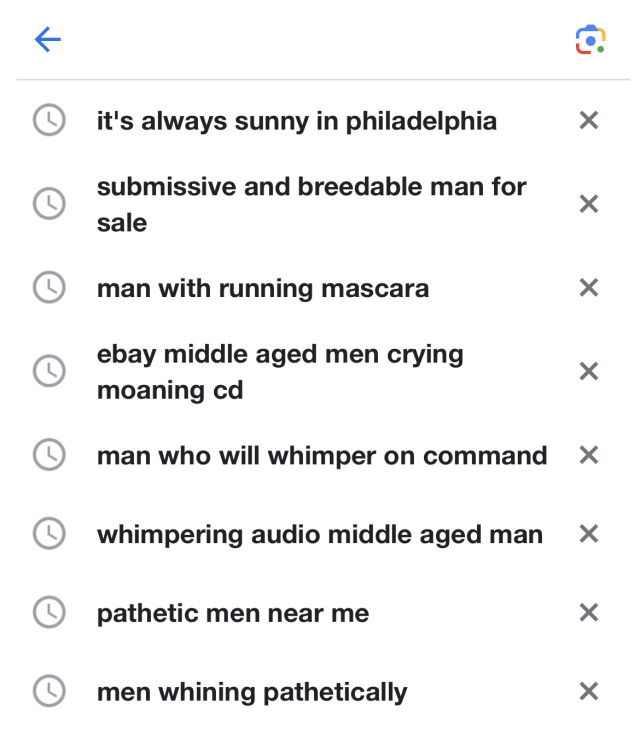This screenshot from a Google search captures an intriguing and unusual set of search queries. In the upper left-hand corner, a blue arrow points to the left, indicating a back navigation option. On the upper right-hand corner, the iconic Google camera icon, adorned in blue, yellow, green, and red, is visible indicating the capability for image searches.

At the top of the screenshot, there is a search result for "It's Always Sunny in Philadelphia," accompanied by a gray clock icon, which may signify that this was a recent search. To the right of this search result is an 'X' button, presumably for clearing the search.

Below, the search history displays a provocative series of searches: "submissive and breedable man for sale," "man with running mascara," "middle-aged man eBay," "men crying, moaning, CD," "man who will whimper on command," "whimpering audio middle-aged men," "pathetic men near me," and "men whining pathetically." Each of these entries is marked with a gray clock icon, suggesting that they are recorded in the user's history.

The screenshot overall is a fascinating glimpse into a series of niche and unconventional search queries, some revolving around submissive behavior and expressions of vulnerability in men.